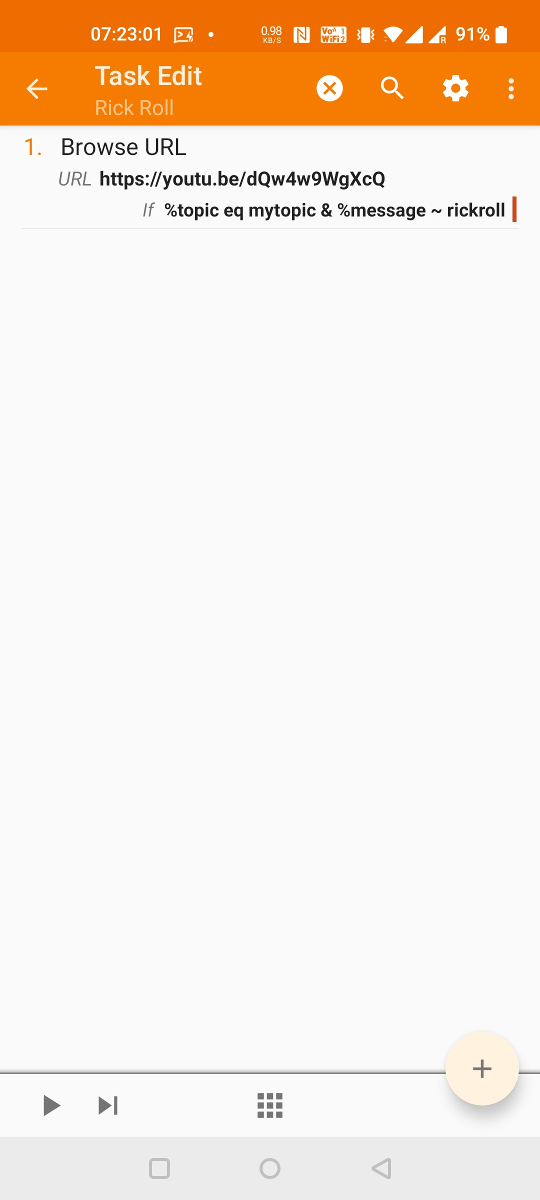The image appears to be a screenshot taken from a smartphone screen that showcases a task or note editing interface. The top of the screen features two horizontal orange bands. The uppermost band is a dark orange, while the slightly thicker, adjacent band below it is a lighter shade of orange. This area displays the current time and various status icons on the right-hand side, including a battery icon indicating 91% power remaining.

Along the lighter orange band, the text "Task Edit" is prominently displayed in white. Just below this, in a very pale orange hue, is the text "Rick Roll." On the left side of this lighter orange band, there’s a white arrow pointing left, possibly indicating a back button. To the right of "Task Edit," several icons are evenly spaced: a white circle with an orange "X" inside it, a white magnifying glass symbolizing search, a white settings icon, and an icon of three vertical dots representing more options.

The section below these orange bands is predominantly white, providing a clean space for content. At the top of this white area, an orange number "1" is displayed, followed by black text reading "Browse URL." Beneath this, the URL "https://youtu.be/DQw4w9WgXcQ" is clearly written. The next line includes italicized text that appears to be part of a code snippet or variable definition: "%topic EQMYTOPIC & %message~rick roll." A vertical orange bar is positioned next to this text block, indicating selection or focus.

Further down within the white space, there is a prominent play button. On the right-hand side, there is a cream-colored oval button with a plus sign inside it. Centrally located is a grid icon consisting of nine gray squares arranged in three rows of three. This content area is enclosed by a thin gray line at the bottom, with a light gray section below it.

This detailed description encapsulates the layout and elements visible in the screenshot, highlighting both functional icons and content-related text.